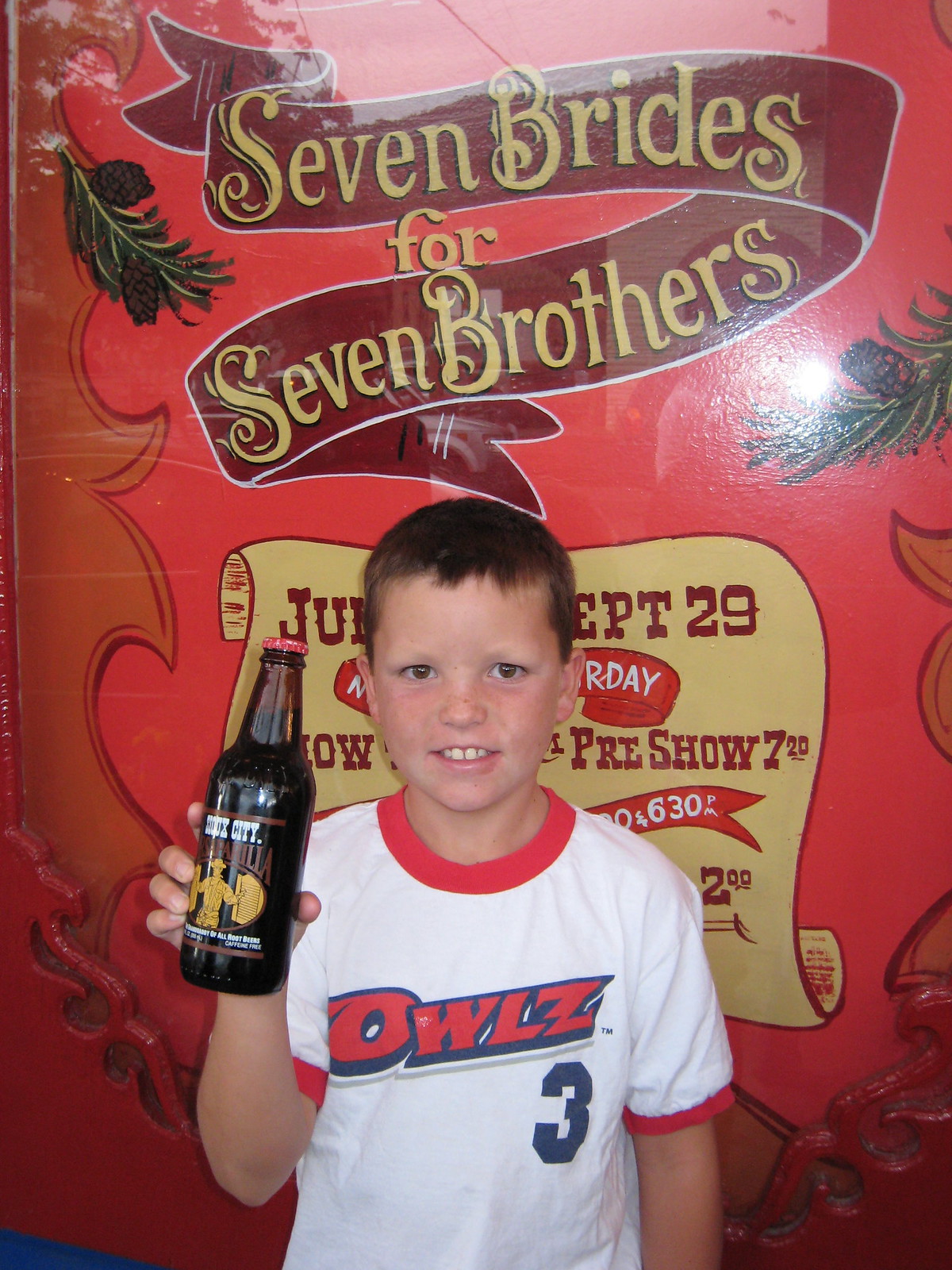In the center of this colored photograph is a young Caucasian boy, approximately 10 years old, with short brown hair and brown eyes. He is dressed in a white t-shirt adorned with red borders around the collar and sleeves. The shirt prominently features the word "OWLZ" in a large red font outlined in blue, along with the number three beneath it. The boy is smiling at the camera, holding an old-fashioned glass soda bottle in his left hand, which is dark brown with a red cap. 

He stands in front of a large, burgundy-colored sign with golden text that reads "Seven Brides for Seven Brothers." The top corners of the image show mistletoe-like leaves, adding a festive touch. Although the majority of the sign is obscured by the boy, glimpses of a schedule can be seen, including details like "September 29th," "pre-show 7:20," "6:30pm," and "$2." The bottle label is partly visible, hinting at "rock city sarsaparilla," featuring an illustration of a cowboy entering saloon doors. This photograph seems to capture the boy's joyful presence at this particular location rather than focusing on the show details behind him.